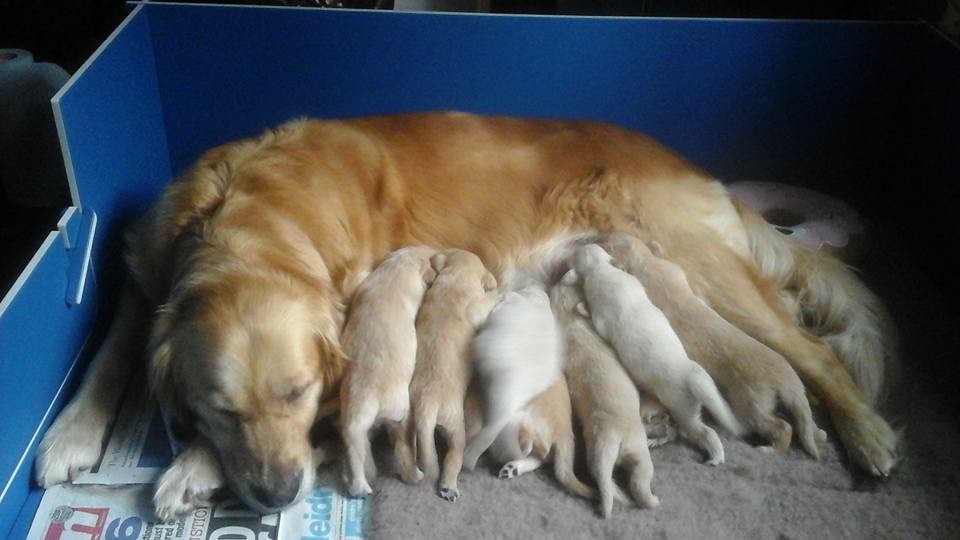In this detailed image, we see a light brown Labrador Retriever mother tenderly nursing her six puppies while lying on her side on an oatmeal-colored carpet. The scene is set within a wooden pen lined with newspaper, with a visible lever near the dog’s head for adjusting the pen's size. The background shows a dark blue half-wall, contrasting with the well-lit room. The puppies vary in color; two on the left are lighter brown, two in the middle are white, and two more on the right are also lighter brown. The mama dog appears serene, drifting off to sleep with her eyes closed, offering a sense of calm and comfort to her clustered offspring. The setup hints at a cozy and organized breeding space, with everything in place for the care and nurturing of the young pups.